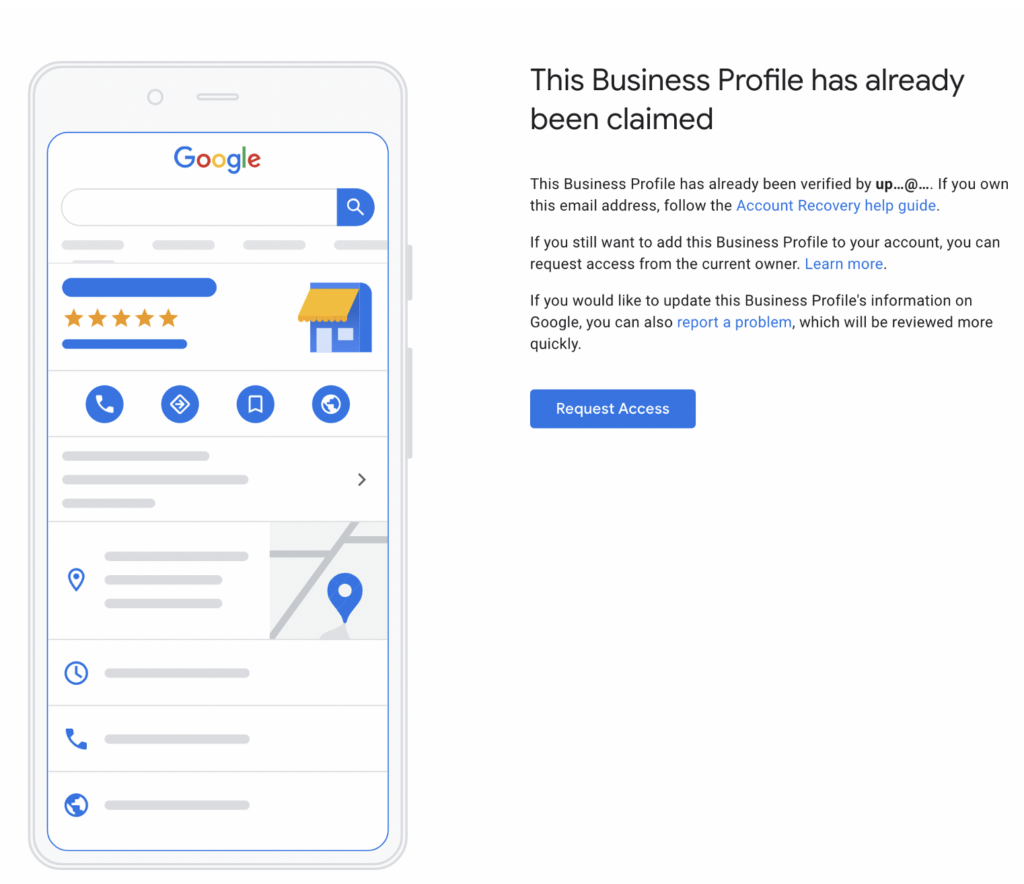**Caption:**

The image depicts a detailed web page screenshot. On the left side, there is an illustration of a smartphone displaying the Google logo in its signature colors of blue, red, yellow, blue, green, and red. Above the logo, there is a search bar accompanied by icons of a phone, a globe, an arrow, and what appears to be a save button. Additionally, there is a placeholder image that resembles the Google Maps interface, featuring a generic gray silhouette of the app with a blue teardrop marker on it.

On the right side of the screenshot, there is a prominent title that reads: "This business profile has already been claimed." Below this, a paragraph explains that the business profile has been verified but does not disclose the associated email address. It advises the user to follow an account recovery help guide if they own the email address in question. Furthermore, it mentions that users wishing to add the business profile to their account can request access from the current owner and provides a link for more information. The paragraph also notes that if users wish to update the business profile information on Google, they can report a problem for faster review. Beneath the text, there is a blue rectangular button labeled "Request Access" in white text.